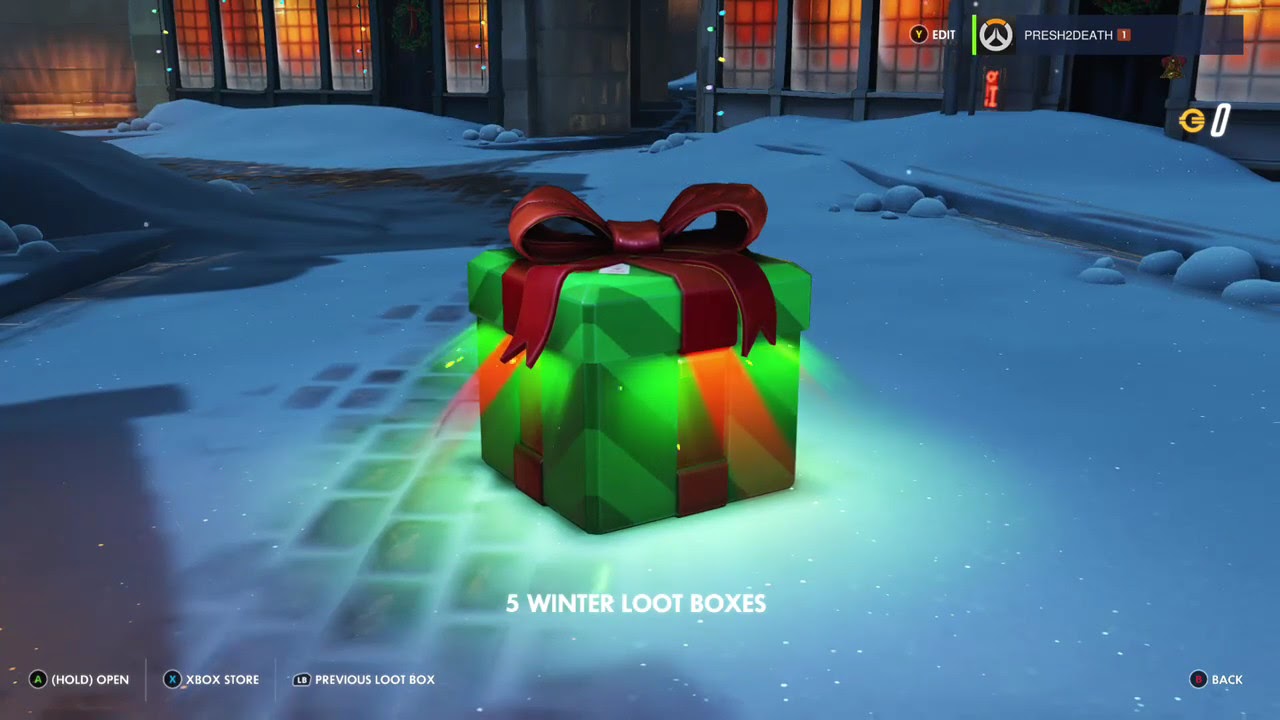The image is a detailed winter-themed screenshot from a video game, showcasing a festive scene. In the background, there is a building adorned with white Christmas lights, and its many windows emit a warm orange glow, creating a cozy ambiance. The ground is covered in snow, and a quaint brick path partially dusted with snow can be seen on the left side of the image.

Prominently featured in the center of the image is a neatly wrapped Christmas present. This green box has light and dark green diagonal stripes, and it is topped with a bright red ribbon and bow. In the lower section of the image, the text "5 Winter Loot Boxes" is displayed in white font, tying into the festive theme.

In the upper right corner, there is informational text that includes the words "Y, Edit" along with a peace sign, "Pre-SH2Death" in white font, and the number "1" enclosed in a small shape that could be circular or rectangular. The lower left corner of the image provides game control instructions: "A, Hold Open," "X, Xbox Store," and "LB, Previous Loot Box." Overall, the scene captures the joy and festivity associated with winter and the excitement of in-game loot boxes.